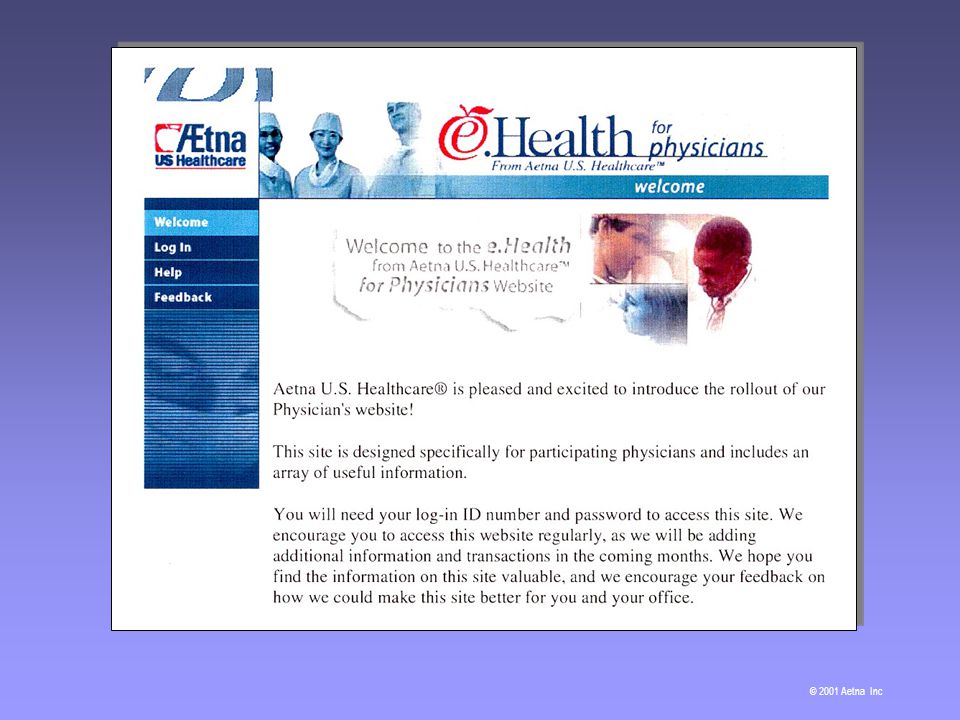Screenshot of an old-fashioned website from Aetna Inc., dated 2001. At the top, the site prominently features the "Aetna U.S. Healthcare" logo, with a banner reading "e-health for physicians from Aetna U.S. Healthcare." The top right corner displays a group of doctors along with a welcoming message. 

On the left sidebar, there are menu options titled "Welcome," "Login," "Help," and "Feedback." The "Welcome" button is highlighted with a different color background. Below the menu is a generic graphic representing a doctor.

The main content area on the right side reads, "Welcome to the e-health from Aetna U.S. Healthcare for physicians website," followed by introductory text explaining the need for login credentials and providing additional information.